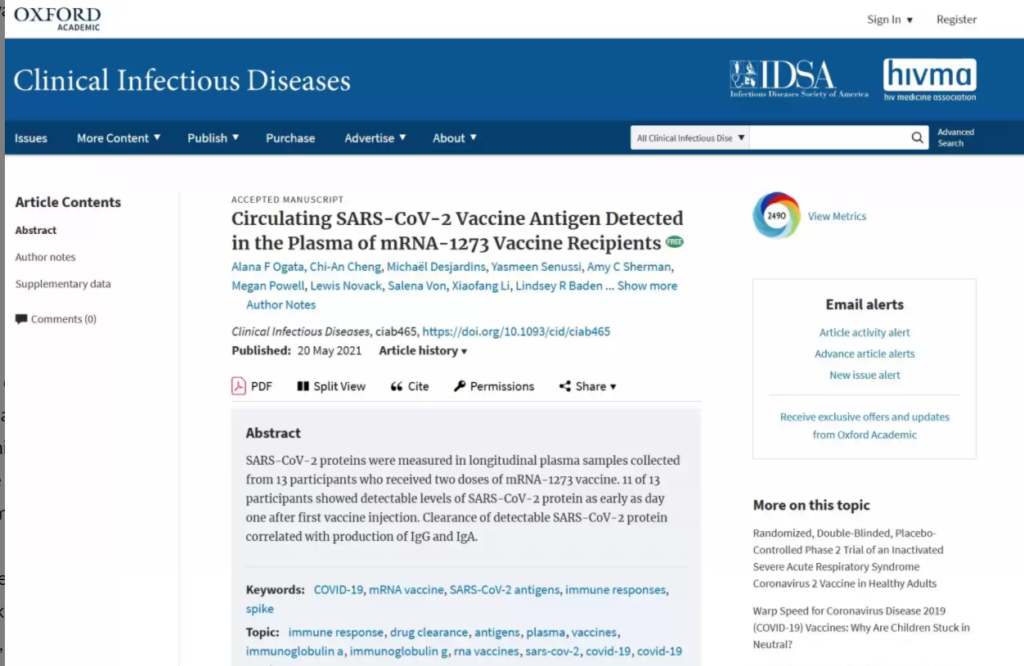A screenshot of the Oxford Academic website is displayed. At the top, there's a white banner with the Oxford Academic logo on the left and "Sign In" with a drop-down menu and "Register" on the right. Directly below this, a blue banner reads "Clinical Infectious Diseases." On the right side of this banner, it lists "IDSA - Infectious Diseases Society of America" and "HIVMA - HIV Medicine Association."

Below the blue banner, there is a darker blue navigation bar featuring tabs labeled "Issues," "More Content" with a drop-down menu, "Publish with Us," "Purchase," "Advertise," and "About" with drop-down menus for each tab. The main section of the page has a white background, displaying several articles.

The highlighted article is titled "Circulating SARS-CoV-2 Vaccine Antigen Detected in Plasma of mRNA-1273 Vaccine Recipients." An abstract summarizes that SARS-CoV-2 proteins were measured in longitudinal plasma samples collected from 13 recipients who received two doses of the mRNA-1273 vaccine; of these, measurements were successful in 11 out of the 13 recipients.